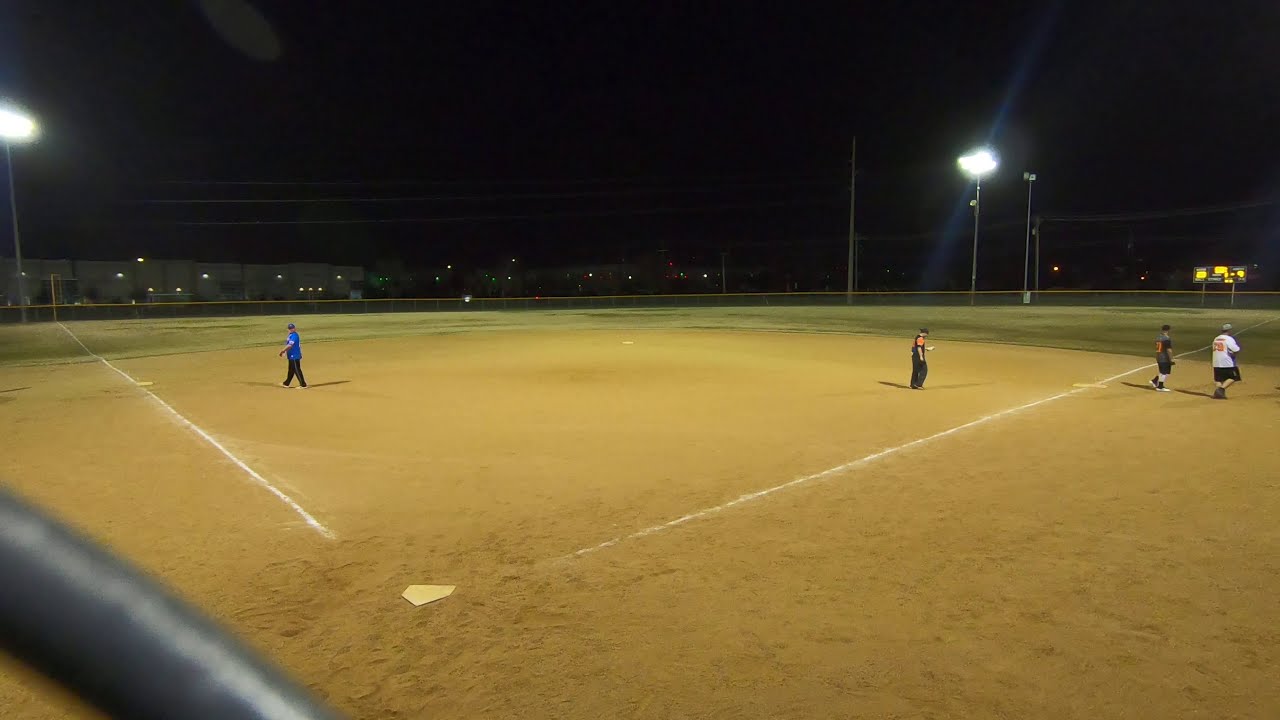The photograph depicts a nighttime scene at a baseball or softball field, brightly illuminated by large spotlights. The sky is pitch black, enhancing the prominence of the well-lit field. Four individuals are scattered across the sandy brown beige baseball diamond. On the left, a person wearing a blue shirt and black pants walks towards third base. Another individual, clad in orange and black, is seen walking towards first base. Near first base, two more people seem to be heading towards the dugout; one wears a white top with orange numbers and black shorts, while the other sports a gray top with orange numbers and black shorts. The individuals are dressed in various colors, suggesting a casual or practice game rather than a uniformed event. Behind home plate, the grass in the outfield appears well-maintained, contrasting with the heavily trodden dirt around home plate. In the background to the right, a blurry scoreboard with yellow digital signs adds to the ambiance of the scene.